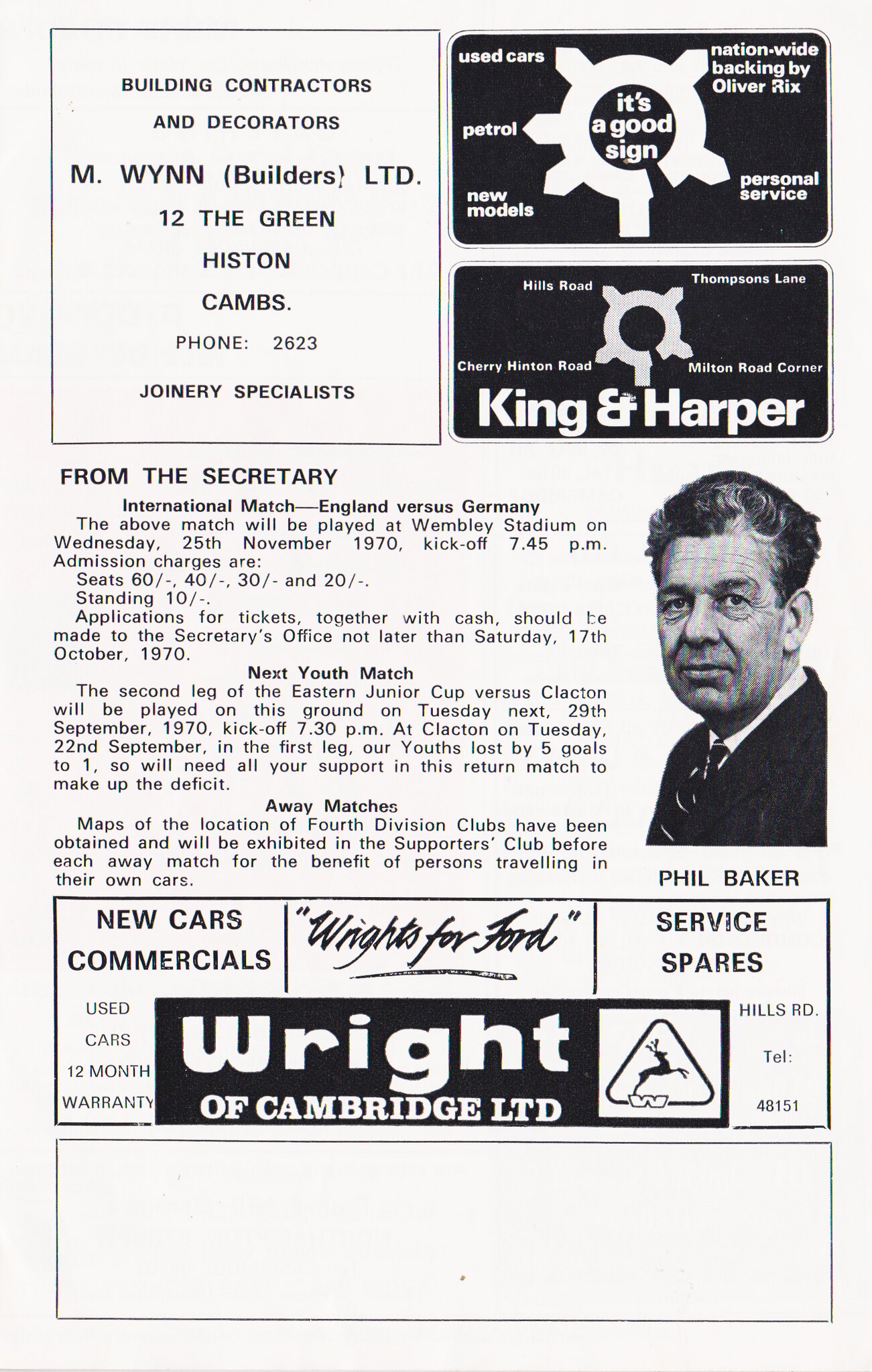This image appears to be a vintage black-and-white page from an old newspaper or magazine featuring multiple advertisements. The layout is vertical and rectangular. At the top left, there's an advertisement for Building Contractors and Decorators: "M. Wynn Builders Limited" with the address "12th and Green, His Stun, CAMBS" and the phone number "2623", highlighting their specialization in joinery. To the right of this is a set of black boxes representing an ad for "King and Harper," which deals in used cars, petrol, new models, and personal service, boasting nationwide backing by Oliver Ricks. Central to the page is a block of text headlined by the secretary's announcement of an international soccer match between England and Germany, including details about the next youth match and away matches. Adjacent to this text stands a black-and-white photograph of an older gentleman in a suit, captioned "Phil Baker," presumably related to the text. Below, another advertisement appears for "Wright of Cambridge Limited," promoting new cars, commercial vehicles, used cars, and service spares, specifically for Ford. The comprehensive layout and blend of textual and visual elements suggest a well-rounded snapshot of the period's commercial and sporting scene.